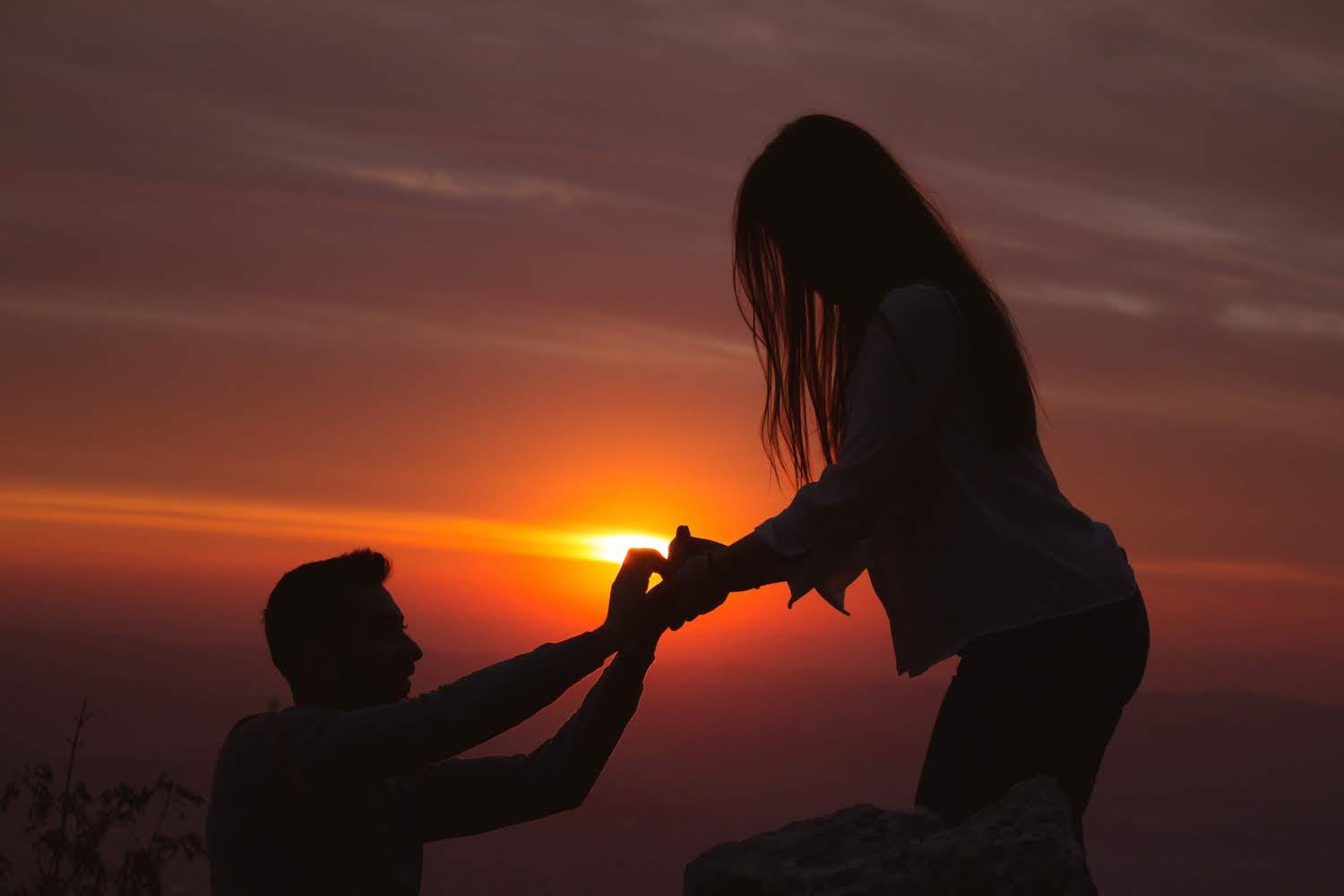Against a stunning sunset backdrop painted in shades of gray, purple, yellow, orange, and blue, a romantic moment unfolds in perfect silhouette on a rocky, elevated terrain, suggesting a mountain or hilltop setting. A man, kneeling on a small rock formation with sparse vegetation around, proposes to a woman standing slightly above him. The woman, dressed in a long-sleeve white shirt and jeans, with her long hair cascading in front of her face, reaches out toward the man, who holds her left hand tenderly in both of his. His short brown hair and gray long-sleeve shirt are subtly outlined by the soft, fading light. In the distance, the horizon is framed by the dark outlines of distant mountains, enhancing the ethereal beauty of this heartfelt scene.